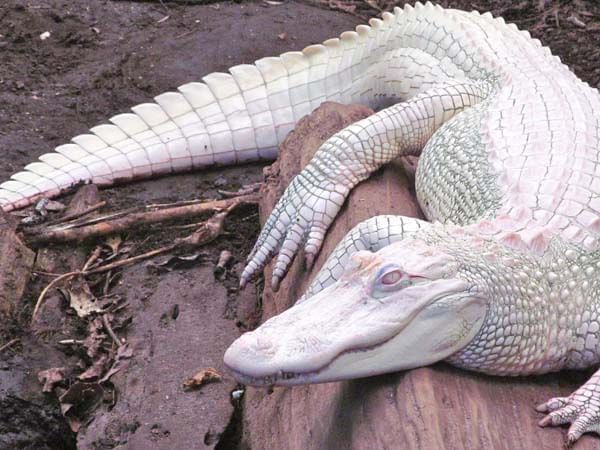This image depicts an albino crocodile, prominently perched on a sizable brown log. The log extends from the bottom right corner of the frame to the middle, providing a perch for the crocodile which is positioned on the right side of the image. The crocodile's body is oriented forward, with its head closest to the viewer but turned to the left, displaying its near-total lack of pigmentation and distinct white coloring. Its scales, arranged in a grid-like pattern, exhibit slight iridescent hues of pale green, pink, and purple, creating a subtle contrast against its overall alabaster appearance. 

The crocodile's tail curves off to the left, and the spiky ridges along its back and tail enhance its textured look. Its mouth, closed but curved in a slight wavy line, and its open, white eye add to the reptilian charm. Detailed scales, each appearing rectangular and pointing slightly upwards along its back and limbs, contribute to the intricate appearance of the reptile. A clawed foot with sharp nails rests in the lower right corner of the frame, further emphasizing the creature's rugged nature.

The background showcases a muddy terrain interspersed with dark brown leaves and sticks, enhancing the natural habitat scene. The image, potentially fitting for a nature magazine, captures this rare and detailed view of a striking albino crocodile basking in its environment.